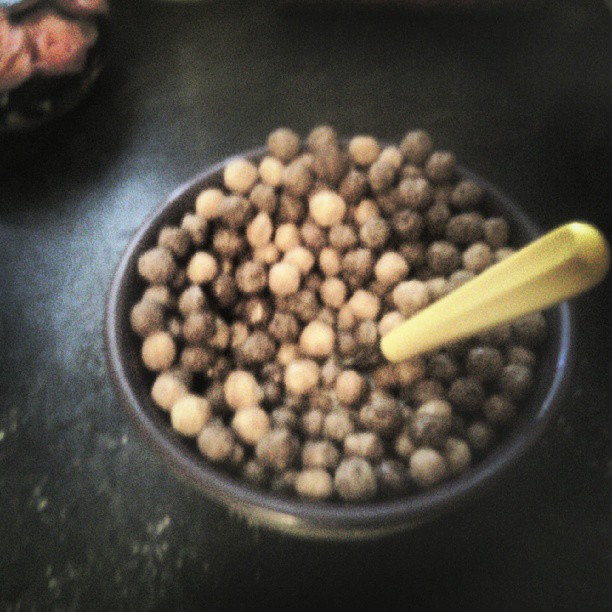The photo depicts a dark, black countertop that appears somewhat shiny, yet also shows signs of damage with speckled white areas. In the upper left corner of the image, there's an unclear object with a pink or peach hue. At the center of the image sits a large, dark-colored bowl, potentially ceramic or plastic. The bowl contains what looks to be a type of cereal consisting of various shades of brown, ranging from light to dark browns. These cereal pieces resemble peanut butter and chocolate Reese's puffs. Inside the bowl is an unusually shaped spoon with a yellow handle, featuring unique grooves. The spoon stands upright, sticking out from the bowl, adding to the overall cluttered yet intriguing scene. While there appears to be milk mixed with the cereal, the image's graininess and blurriness make it hard to confirm this detail with certainty.